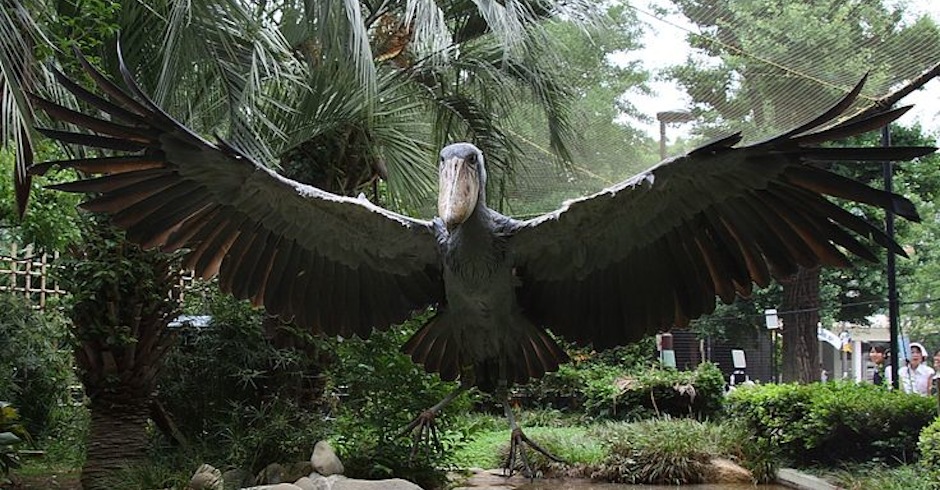The image captures a gigantic bird, likely resembling a stork or pelican, with an enormous wingspan and a massive beak. Its plumage is primarily a mix of gray, black, and white, with black feathers prominently at the tips of its wings. The bird appears to be gazing slightly off-camera while stretching its wings fully, giving a clear view from underneath. The backdrop reveals lush, green foliage including trees and palm fronds, suggesting a lush habitat, and it's enclosed within netting, indicating a zoo setting. In the background, two spectators are visible behind a caged area, observing the bird. A fireplace, currently unlit, is also present in the scene, adding a curious detail to the overall setting.